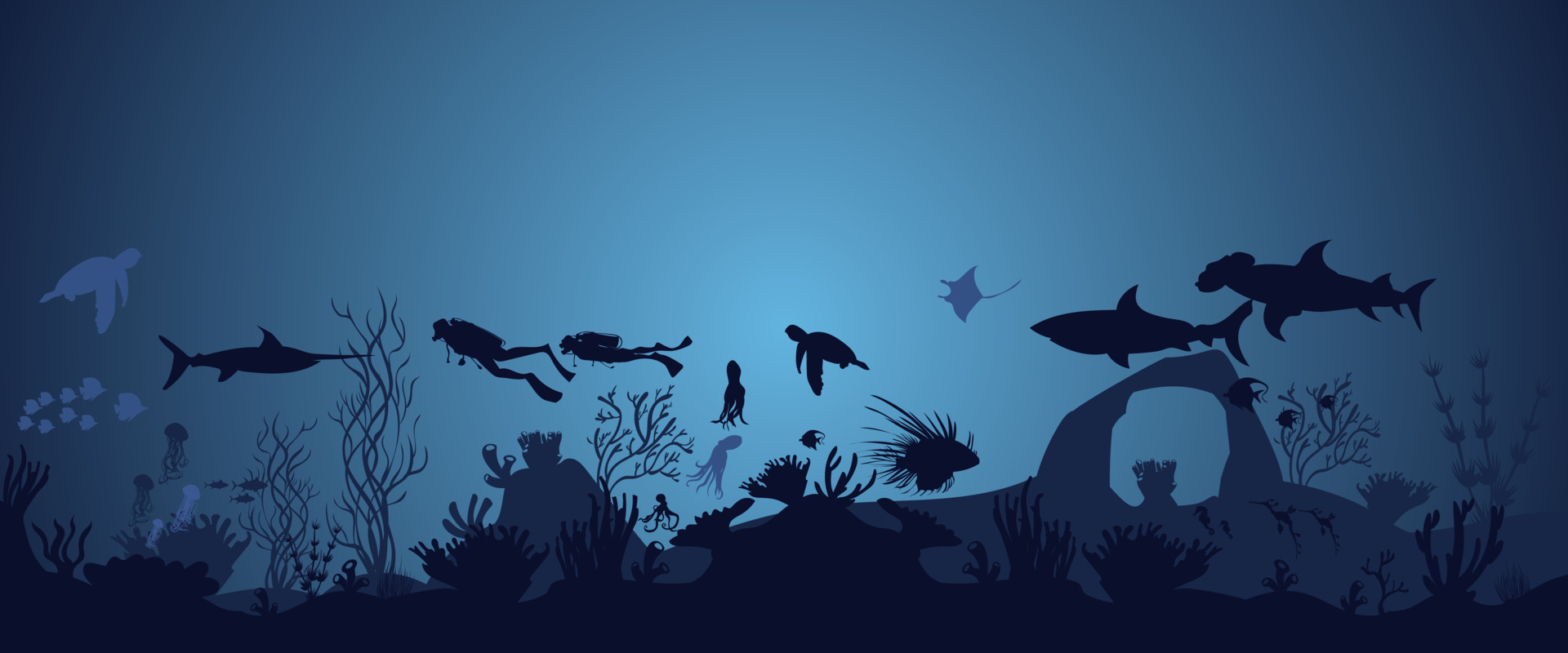This highly detailed rectangular illustration captures a vibrant underwater scene, dominated by shades of blue and black. In the center left, two scuba divers in full gear explore the aquatic world, while a large swordfish gracefully points towards them. Above, on the upper left, a lighter-colored turtle swims leisurely, with a school of light blue fish gliding beneath it. Various sea creatures populate the illustration, including two or three octopi, a spiked fish, a manta ray, and both a great white shark and a hammerhead shark on the right side, adding to the diversity of marine life depicted.

The seafloor at the bottom of the image is portrayed in darker hues of gray and black, adorned with anemones, vegetation, and other typical ocean floor shrubbery. The water's color gradient transitions from a lighter blue in the midsection to darker blues on both the left and right sides, creating a dynamic backdrop. Small silhouettes of underwater plants and landscapes can also be seen, adding further depth to the scene. Notably, amidst the aquatic life, there are a couple of distinctive white spots to the left, potentially representing fish or other items. This intricate painting beautifully illustrates the bustling and varied ecosystem beneath the ocean’s surface.